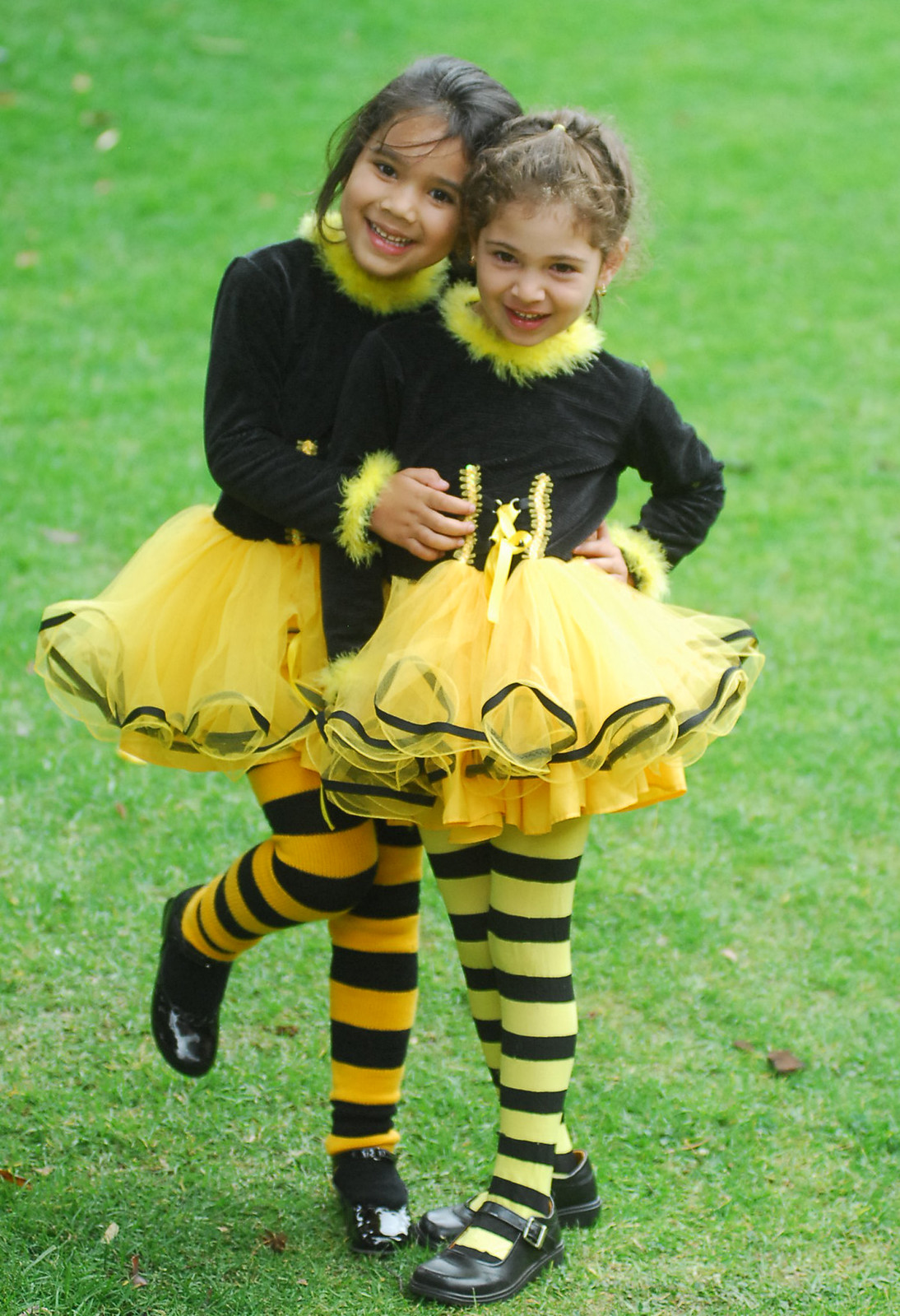The image captures two young girls, probably around five to eight years old, standing and hugging amidst a verdant green field strewn with leaves. Both are dressed in adorable honeybee costumes, featuring black tops with yellow furry collars, yellow skirts, and knee-high socks adorned with yellow and black stripes. They sport matching black dress shoes. The girl in the foreground wears a yellow dress with a black top and yellow furry collar, complemented by striped stockings. She has a touch of brown in her hair and is joyfully laughing at the camera. Her friend, who has darker black hair, stands behind her, hugging her with her left arm and placing her right hand on the first girl's belly. She rests her head on the shoulder of the girl in the foreground and raises her right leg while standing on her left. Both girls are smiling broadly, sharing a moment of happiness and camaraderie.